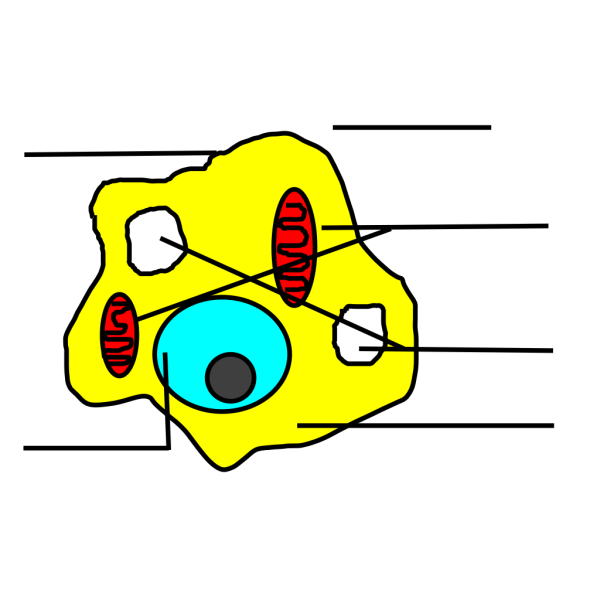The image is a digitally rendered cartoon illustration depicting the various parts of a cell or a microorganism, set against a solid white background. The cell itself is an amorphous yellow blob with a black border. Inside this yellow shape, there are several distinct elements: two red ovals with black squiggly lines, two irregular white circles with black outlines, and a larger blue circle with a black border containing a smaller dark gray circle, reminiscent of an eyeball. Black lines and bars are scattered around and pointing to these components: four lines on the right side with two of them extending from the cell’s center, and two lines on the left side, where only one directs towards a part of the cell. The combination of these colorful shapes and directional lines creates a detailed and intricate illustration of cellular components, providing a visually engaging representation of biological structures.